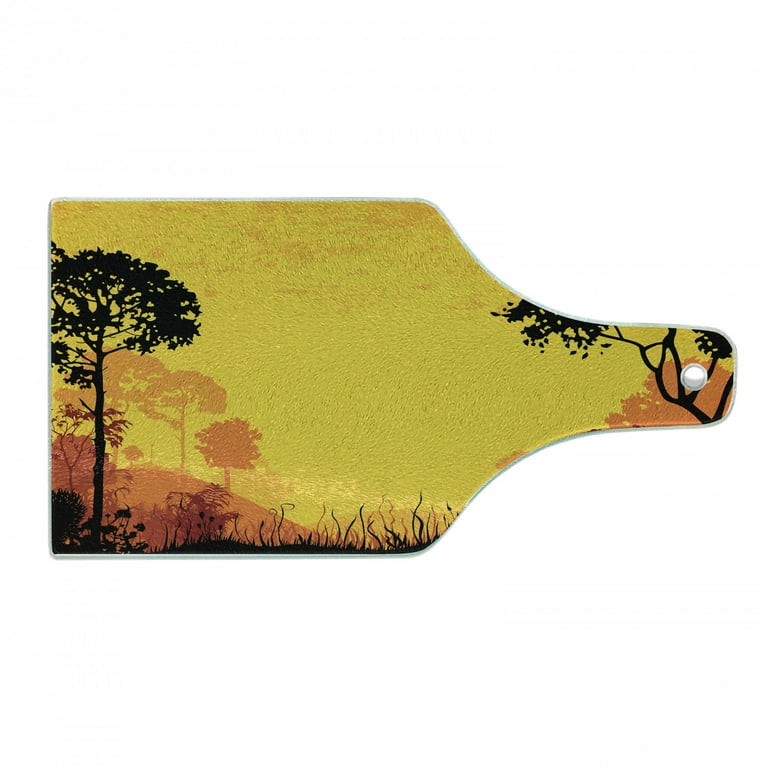This image depicts a uniquely designed cutting board set against a solid white background. The cutting board, which could also be taken for a paddle, features an intriguing shape that consists of a narrow, rectangular handle tapering outwards into a wider, roughly square or rectangular cutting surface. This handle is positioned towards the right and includes a circular cutout near its tip, presumably for hanging purposes.

The cutting board showcases an elaborate forest scene painted on its surface. Dominating the left side is a tall, thin black tree shaded with black leaves, while smaller black grasses or weeds grow at its base. The backdrop transitions from light yellow to deeper hues, including light orange and red, ultimately leading to black in the foreground, which suggests layers of hills and foliage. The scene also includes hills painted in shades of orange and brown, indicating a layered landscape that becomes darker and more defined as it approaches the foreground.

On the right side, near the handle, brown tree branches with black leaves encircle the circular cutout, adding a rustic touch. Overall, the primary background color of the cutting board appears to be a deep yellow that enhances the vivid details of this picturesque forest landscape.